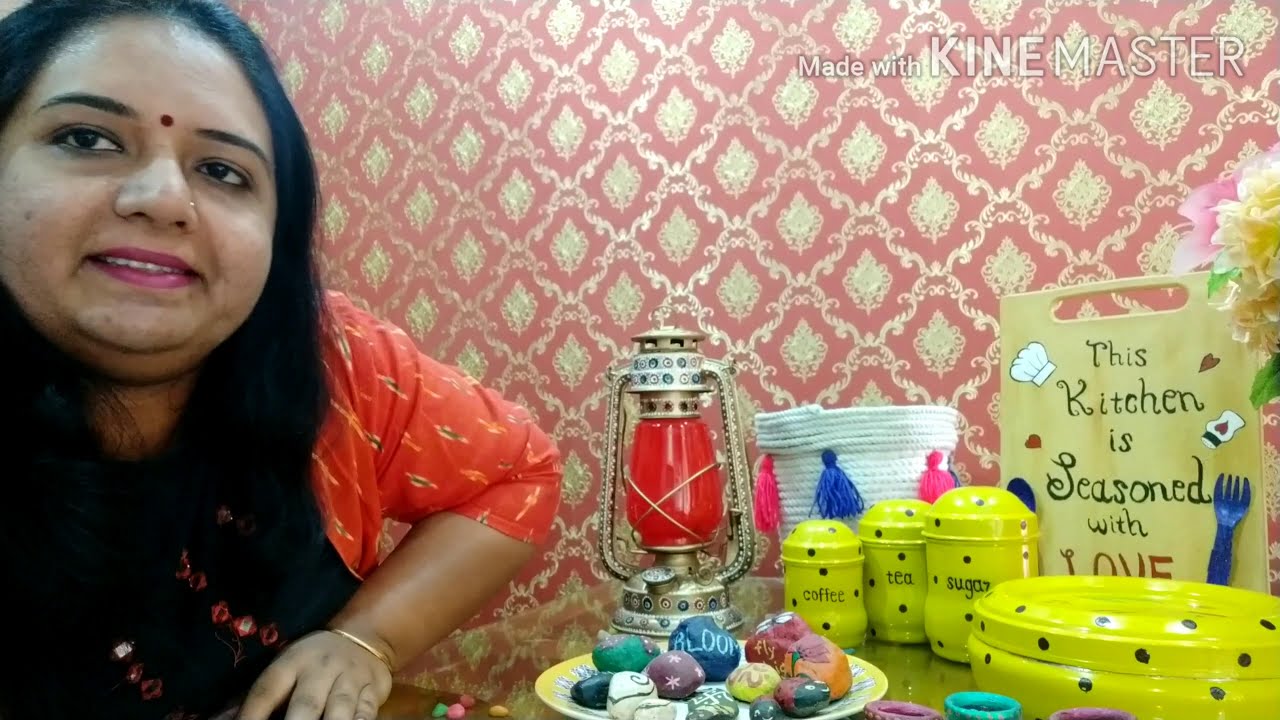This is a detailed photograph taken inside a cozy, vibrantly decorated home. On the left side of the image, an Indian woman with a round face and light brown skin sits at a table. She has long, black wavy hair that flows past her shoulders, and she wears a red and black outfit adorned with a bindi on her forehead and pink lipstick. Her red shirt features little yellow stripes and is paired with a black vest decorated with red flowers. A gold bracelet gleams on her wrist. 

To her right is a small, heavily decorated table overflowing with colorful items. Among them are four yellow canisters with black polka dots labeled for coffee, tea, and sugar, a red lantern, and a plate with painted rocks or possibly sweets. A wooden sign shaped like a cutting board stands prominently, reading, "This kitchen is seasoned with love." 

In the background, the wall is covered with an elaborate pink and gold-patterned wallpaper, creating a warm and inviting ambiance. In the upper right corner of the photograph, the watermark "Made with KINEMASTER" is visible.